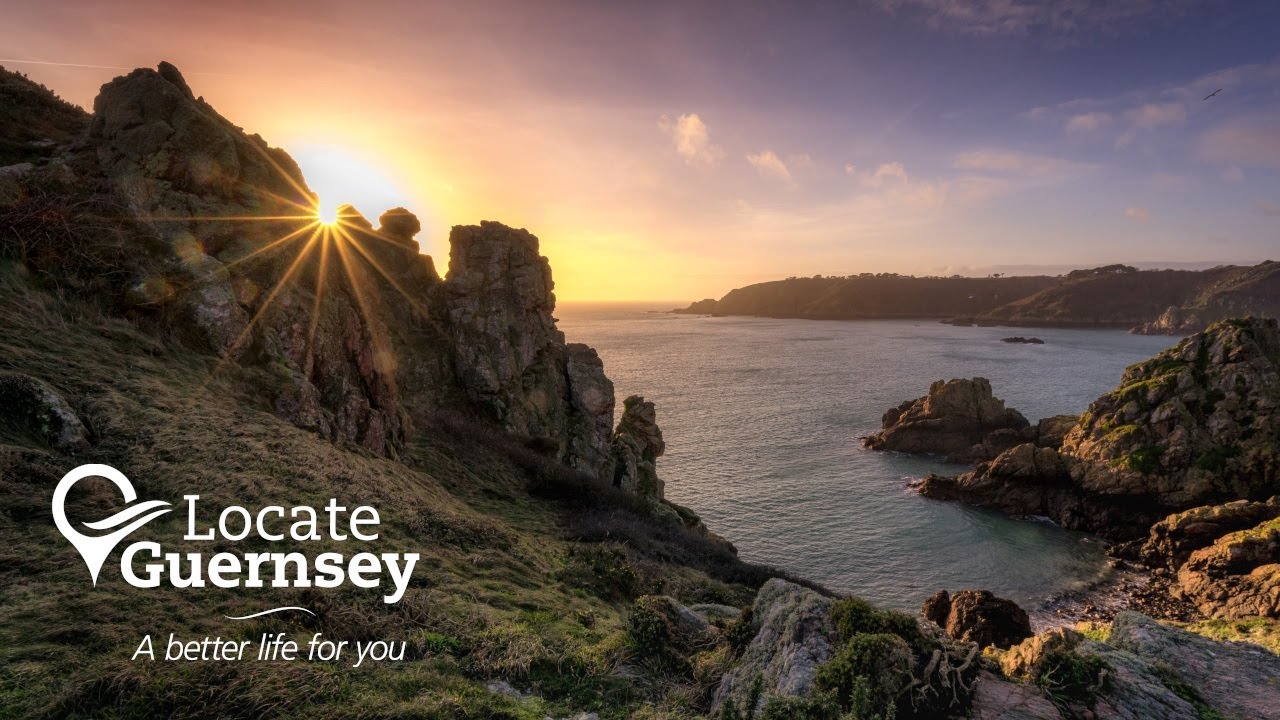This captivating photograph serves as an advertisement for Locate Guernsey, featuring the tagline "A better life for you" prominently displayed in white lettering in the bottom left corner. Set during a sunlit transition—either sunrise or sunset—the scene showcases the serene beauty of a mountainous landscape meeting the water, which could be an ocean or a large lake. The sky exhibits a muted palette of blues and pinks with a scattering of clouds, enhancing the tranquil ambiance. On the left-hand side, the sun's rays peek dramatically through a rugged rock formation, casting a picturesque glow over the water and the moss-covered rocks that extend into the scene. The composition, rich with greenery, rock formations, and reflective, crystal-clear water, evokes a sense of calm and natural beauty, reminiscent of landscapes found in regions like Ireland or Scotland.